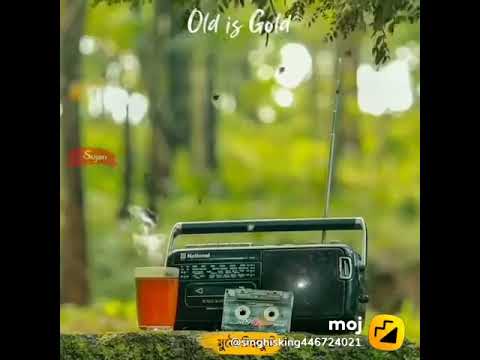The image depicts a vintage black cassette radio player, often referred to as a boom box, which has a long horizontal design and a prominent antenna on the right-hand side. The boom box also features a handle for portability. In front of the radio, leaning against it, is a gray cassette tape. To the left of the cassette player is a transparent glass filled with a reddish-orange liquid. The scene appears to be situated outdoors during the daytime, with a blurred forest green background that sets a nostalgic tone. White text at the top of the image reads "old is gold" in a handwriting-style computer font. There is additional text and a small emoji in the bottom right corner, further enhancing the image's vintage commercial feel. The image itself is bordered with vertical black bands on the left and right, giving it a framed appearance. The entire composition rests on what looks like a moss-covered stone, enhancing the retro and timeless atmosphere of the picture.